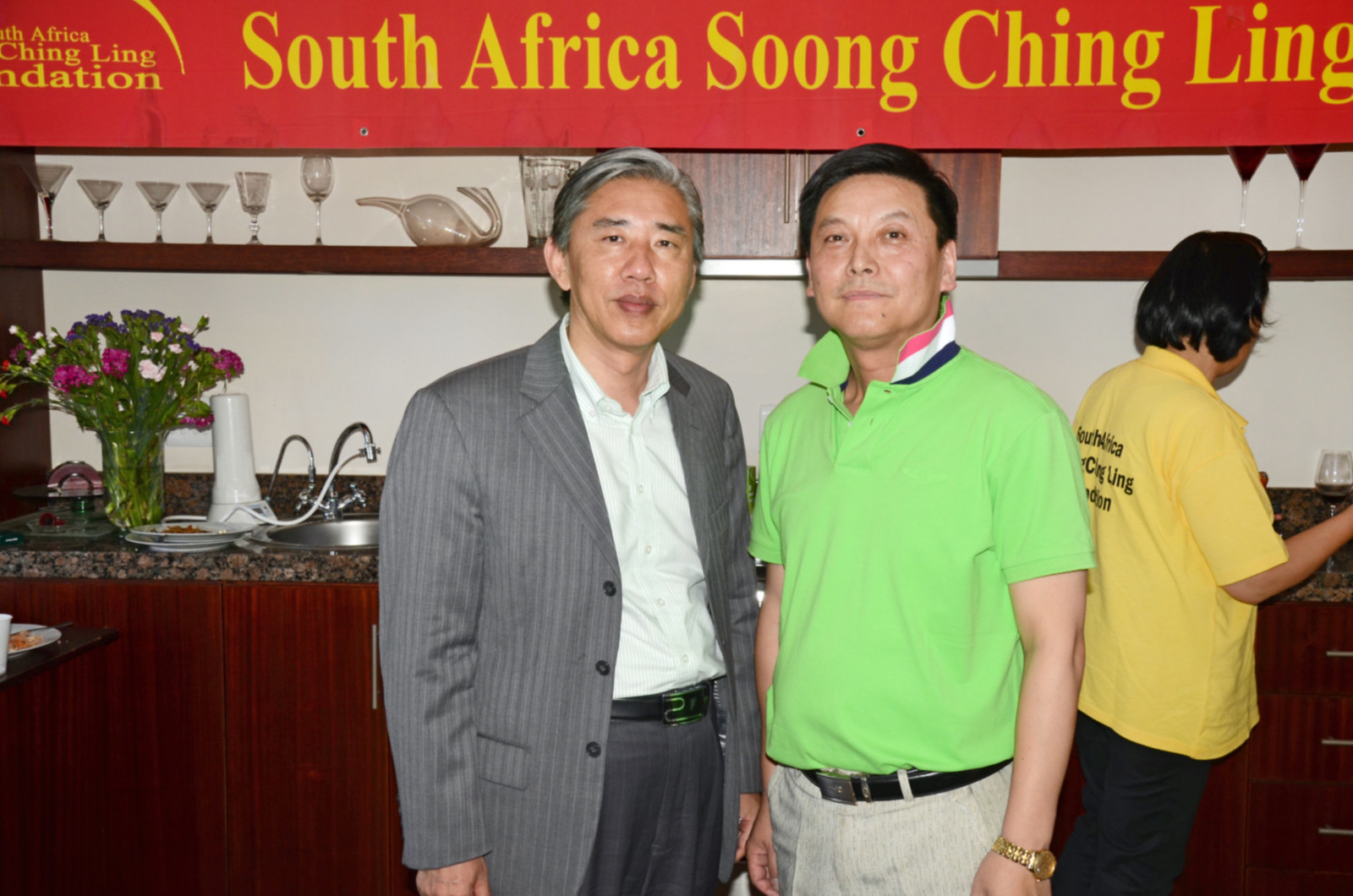In the photograph, three individuals are present, prominently set against a detailed indoor backdrop. Two men stand facing the camera. The man on the left wears a gray-striped sports coat over a white undershirt, accompanied by gray slacks and a belt, giving him a distinguished appearance with his gray hair. To his right, a younger man with black hair is dressed in a lime green polo shirt with a colorful white, pink, and blue collar, paired with khaki pants and a black belt, accentuated by a gold watch on his wrist. The third individual, positioned further to the right with their back turned, is wearing a yellow shirt with black writing and black pants, leaving their gender ambiguous due to their long black hair and unobscured face.

The environment is distinctly furnished with wooden cabinets and a marble countertop behind the three figures. On the left side of the backdrop, a bouquet of flowers adds a touch of color and life. A plate and a sink are visible on the countertop, suggesting a functional kitchen or bar area. Above the countertop, a shelf holds an array of wine glasses and various other glass objects, contributing to the setting's elegant ambiance.

At the top of the image, a striking red banner with yellow lettering reads, "South African Tsun Ching Ling." To the left of the banner, additional text references the Tsun Ching Ling Foundation, highlighting the context of the image. This setting, combined with the attire of the individuals, suggests a formal event or gathering associated with the foundation.